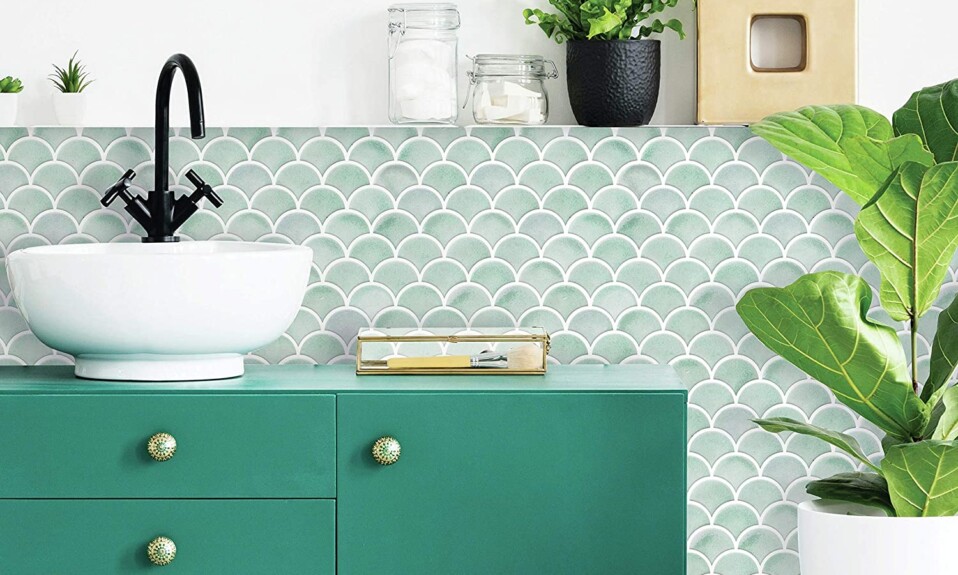The image depicts a modern bathroom with a striking, artistic design. The wall features a unique, aqua-colored, half-circle tile pattern reminiscent of mermaid scales, which adds texture and visual interest. Above the tiles, a white wall contrasts against the colorful backdrop. Below this, a dark aqua green bathroom cabinet becomes the room's centerpiece, adorned with three goldish knobs placed on the top, bottom, and right side. Atop the cabinet sits an elegant bowl-style white sink paired with a sleek black faucet. 

Off to the side of the cabinet rests a notable fiddle leaf fig plant in a white pot, adding a touch of natural greenery. On the bathroom cabinet, there is also a clear box lined with gold, holding a tan object. Beyond the main fixtures, an overhead ledge runs parallel to the tiles, hosting a variety of decorative and practical items. From left to right, the ledge accommodates two small white pots with plants, two clear glass jars containing makeup wedges and cotton balls, a black planter with a small green plant, and finally, a decorative tan wooden box with a cutout center. This carefully curated arrangement emphasizes both functionality and aesthetics, making the bathroom a harmonious blend of utility and style.